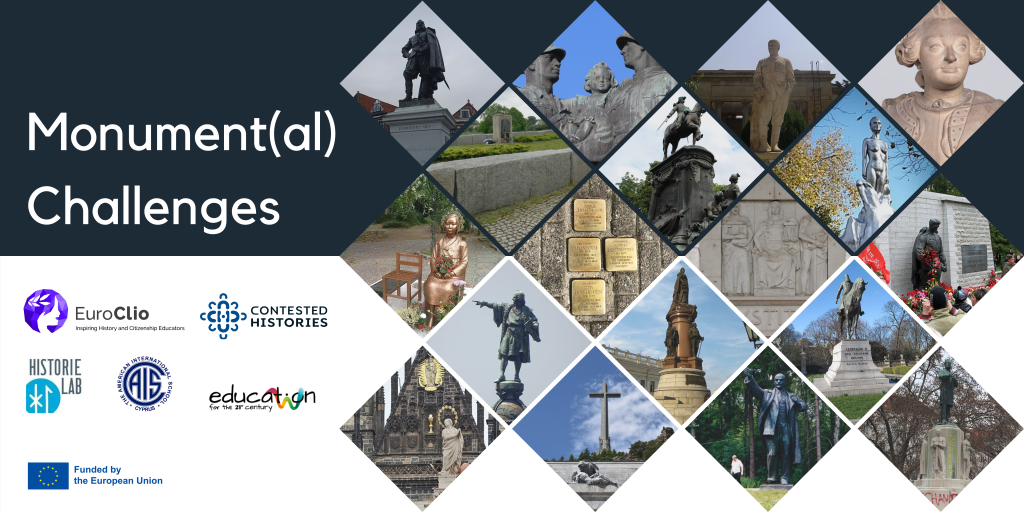This is a rectangular advertisement poster featuring a collage focused on historic monuments. Dominating the upper left-hand corner is the title "Monument(AL) Challenges" in white text against a dark blue backdrop. Below this title, a series of sponsor logos are distinctly displayed, including "Euroclio," "Contested Histories," "Education for the 21st Century," "HistoriLab," and the note "Funded by the European Union." The central portion of the poster is occupied by a diamond or square-shaped grid, each section showcasing a photograph of various statues and monuments from around the world, likely Europe. The monuments are made of different materials, such as bronze, gold, and cement, and exhibit a range of colors, from golden hues to tarnished greens. Included in the images are numerous statues of individuals, including two men on horseback and a grand cross, suggesting religious significance. The intricate collection of these historic pieces invites the viewer to reflect on the diverse and contested histories they represent.